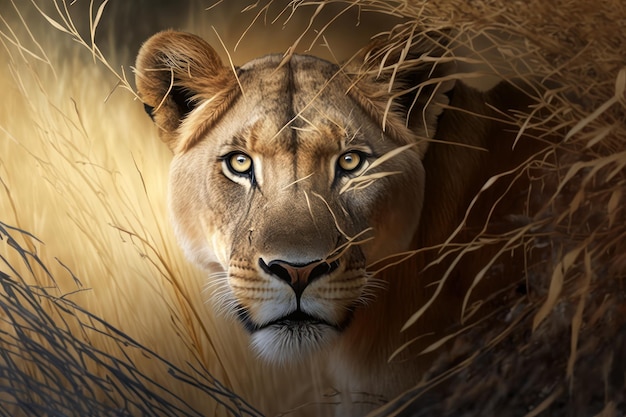This detailed artwork presents a close-up of a female lion's face, centrally positioned, giving the illusion of a lifelike encounter. The lion's fur is predominantly light brown, with distinctive white markings around its mouth, nose, and eyes. The eyes, a pale yellow, convey an alert and focused expression. A subtle black stripe runs from the top of its head down to its nose, and hints of black are also visible in its ears. The image is intricately detailed, capturing every tiny hair to enhance its realism. Surrounding the lion are strands of yellowish-brown grass, some of which bend and fall in front of its face, with a few strands seemingly entangled in its fur. The background features a mix of this tall grass, becoming blurred and out of focus behind the lion, which adds depth to the scene. There is also a patch of darker grass in the bottom left corner, enriching the image's textural complexity.